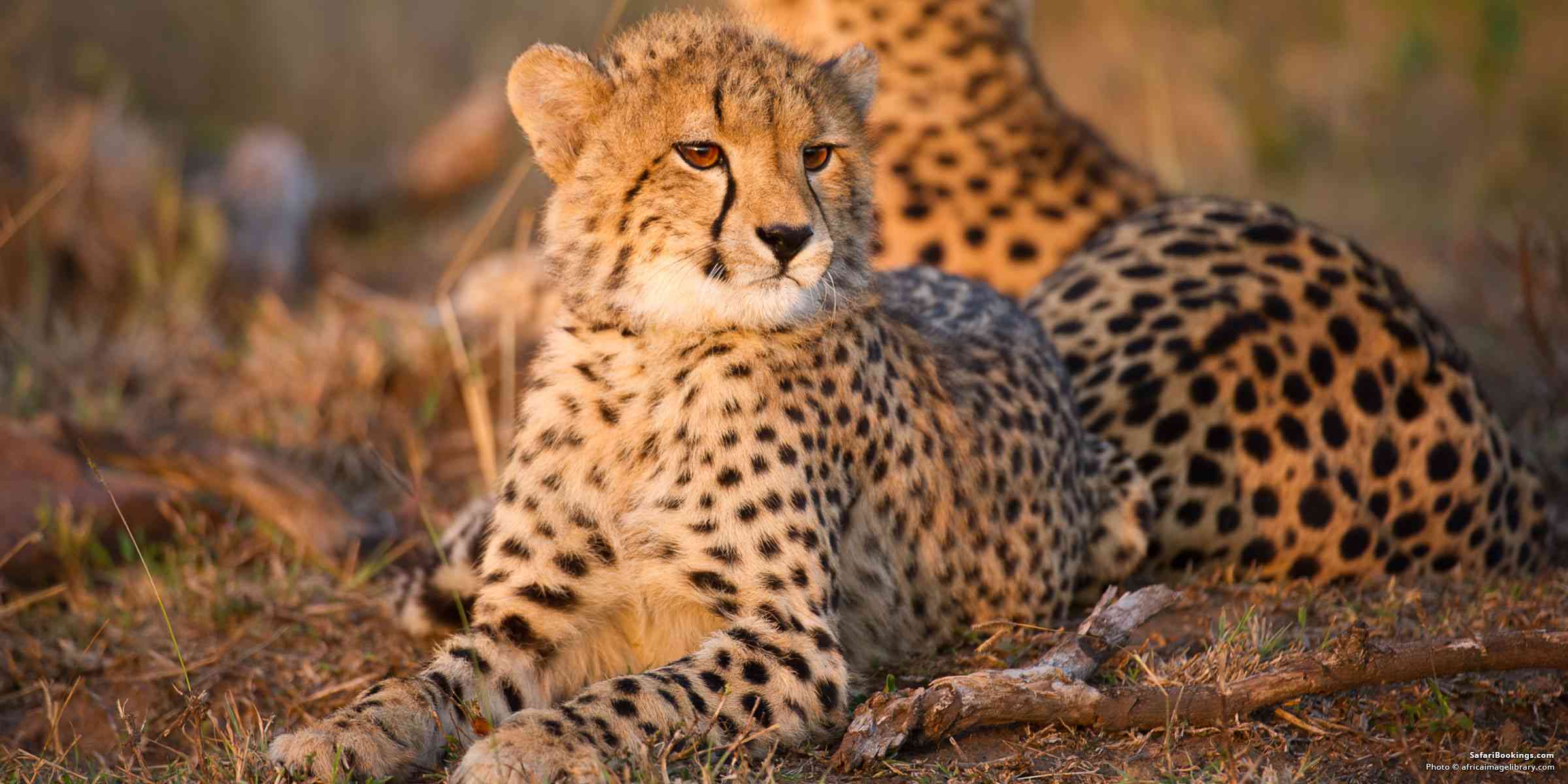In a captivating landscape-oriented photograph taken closer to evening, a baby cheetah with light brown fur adorned with black spots sits alertly in the center, gazing pensively to the right. The cub's striking amber eyes, black nose, and facial stripes are in sharp focus, emphasizing its youthful elegance. It sits amidst mostly dry, sparse grass and some gray, broken-off tree branches. Behind the cub, a larger cheetah—presumably its mother—rests, slightly out of focus, blending into the earthy tones of their environment. The background cheetah faces the opposite direction, its spotted coat and relaxed posture adding context to the familial scene without diverting attention from the engaging presence of the cub.